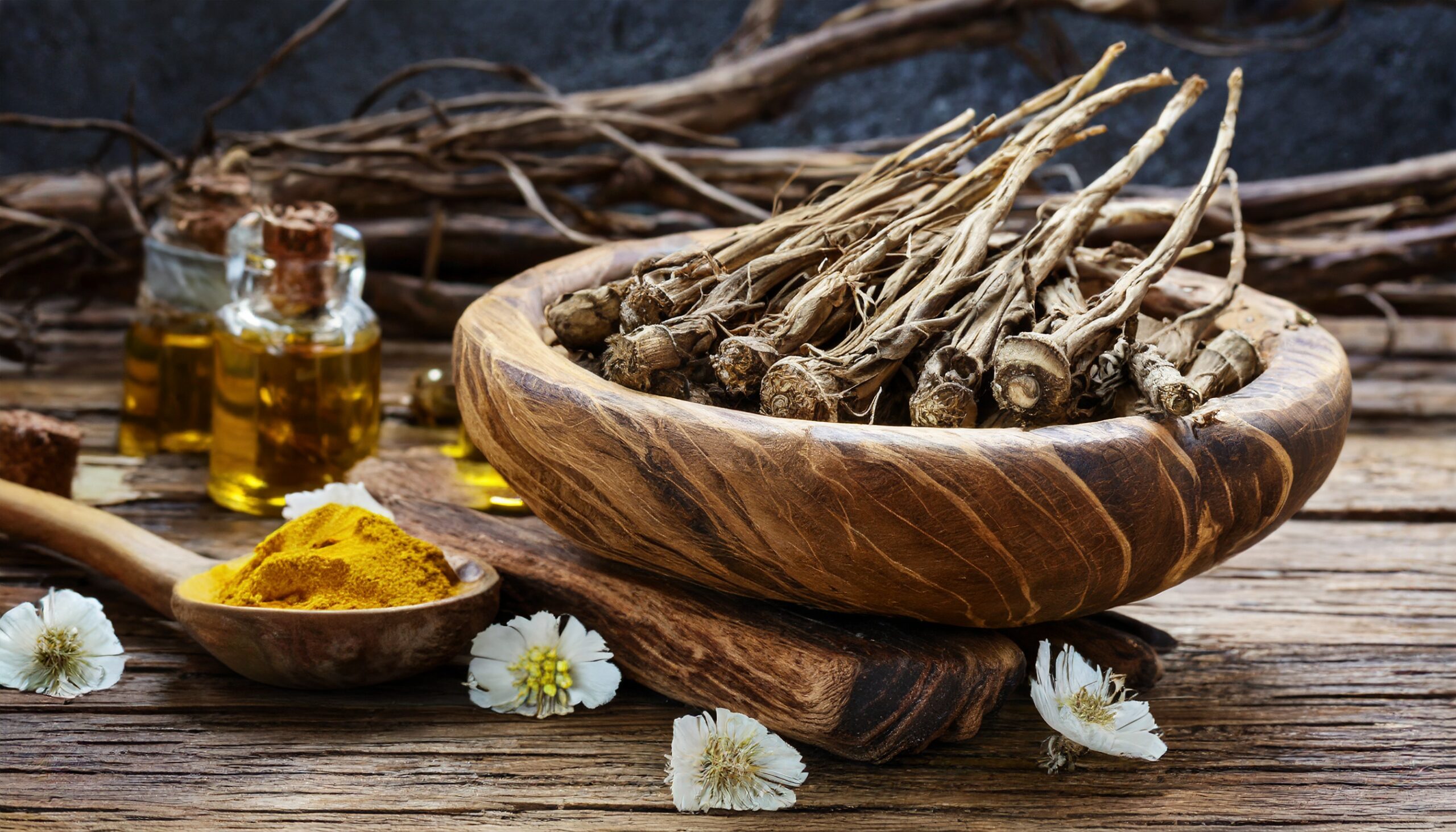In this color photograph, a large wooden bowl, resting on a wooden plank, contains a series of long, stick-like herbs arranged neatly beside each other. A wooden spoon filled with a heaping pile of turmeric-yellow seasoning lies adjacent to the bowl. The scene is set on a wooden surface adorned with four white flowers with yellow centers. In the slightly blurry background, two small glass bottles filled with an amber-colored liquid and sealed with cork stoppers are visible. A collection of longer branches and sticks, along with a bluish-gray backdrop, further emphasize the rustic and natural ambiance of the photograph. The exact nature and purpose of the herbs and sticks in the wooden bowl remain ambiguous, adding an element of mystery to the composition.